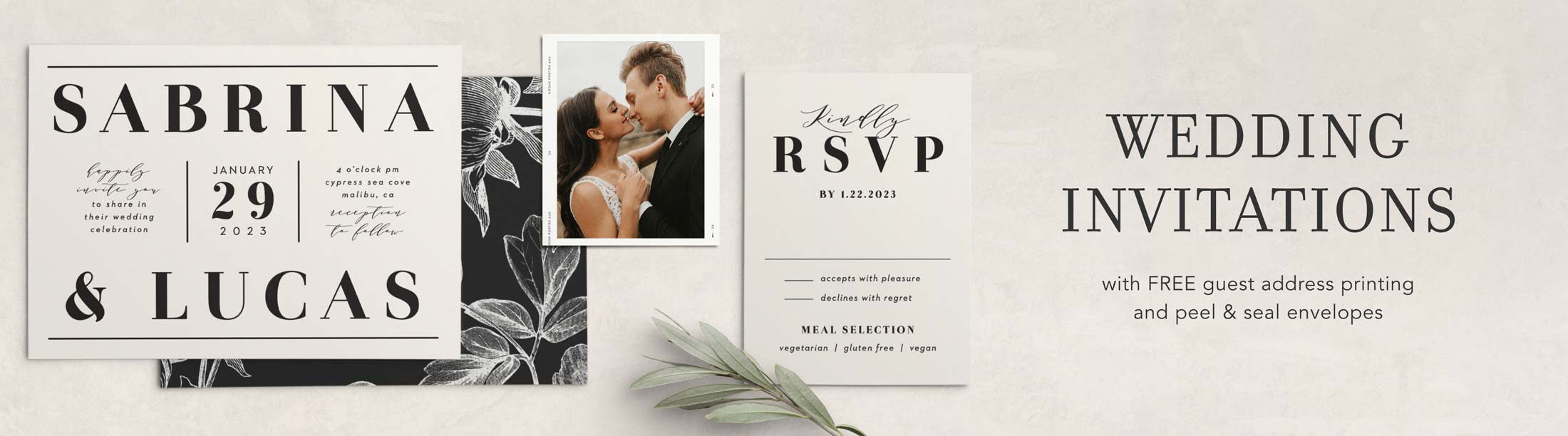The image is an advertisement for wedding invitations set on a pale background. Dominating the left half of the advertisement is a save-the-date card for Sabrina and Lucas, scheduled for January 29th, 2023. The card features black text on a cream background and includes a photo of the couple, Sabrina and Lucas, in an affectionate embrace, gazing happily at each other. This romantic image is accompanied by floral elements in the background, adding to the elegant ambiance. Beside the couple's photo is a small RSVP section requesting responses by January 22nd, 2023. The right side of the advertisement highlights the service offerings, stating, "wedding invitations with free guest address printing and peel and seal envelopes," all in black text. Additionally, a piece of greenery, possibly eucalyptus, decorates the bottom edge of the advertisement, enhancing its sophisticated and natural appeal.